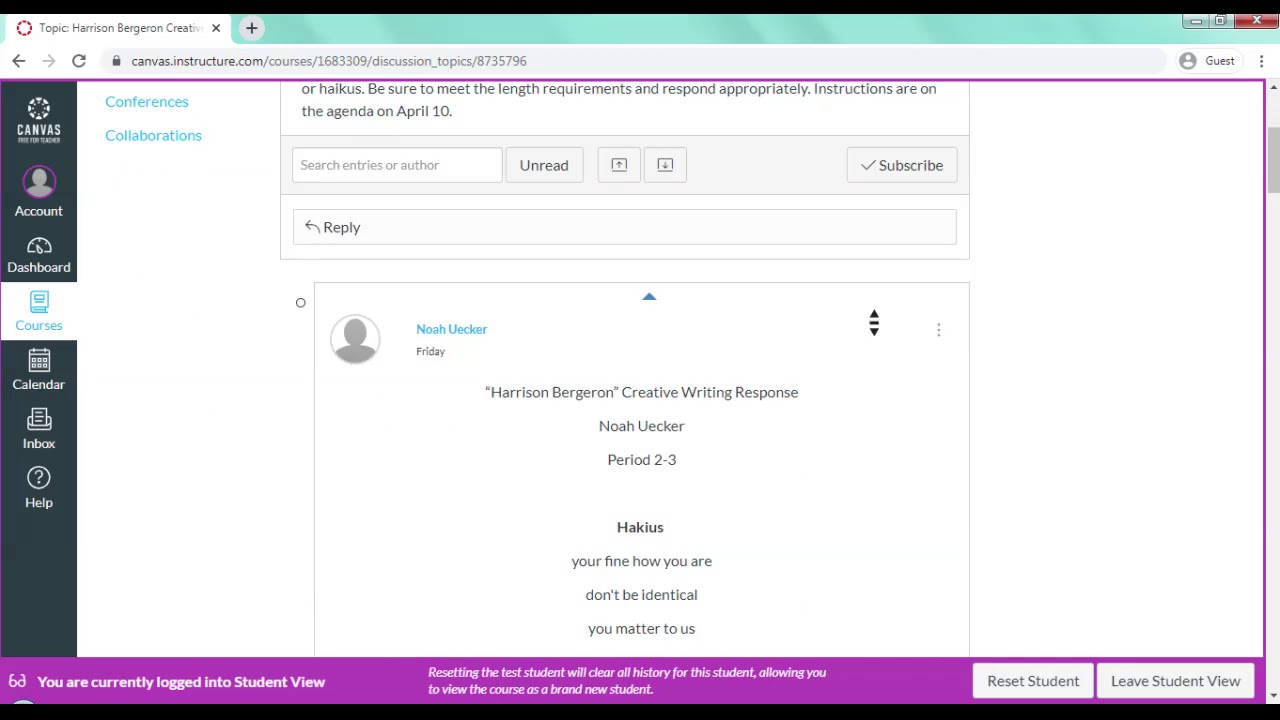This horizontal screenshot showcases a browser window with a webpage open on a white background, featuring the educational platform Canvas. At the top, a speckled light aqua banner is framed by thin black borders. The single open tab reads "Topic Harrison Bergeron Creative," with the web address "canvas.instructure.com" displayed next to a secure lock icon, flanked by a back arrow, refresh button, and a "Login as Guest" button.

The main content area is framed by a thin purple border with a vertical scrollbar labeled "Canvas." The sidebar contains icons for "Account," "Dashboard," "Courses," "Calendar," "Inbox," and "Help." The "Courses" tab is highlighted in light blue, and immediately below the address bar, "Conferences and Collaborations" is noted. 

Prominently, a post by a user named Noah Uker is displayed, titled "Harrison Bergeron Creative Writing Response Noah Uker period 2-3." The post features a haiku: "You're fine how you are, don't be identical, you matter to us."

At the lower edge of the image, a purple bar indicates, "You are currently logged into Student View. Resetting the test student will clear all history for this student, allowing you to view the course as a brand new student." Two buttons, "Reset Student" and "Leave Student View," are positioned in the lower right corner. The screenshot is enclosed with a thin black border mirroring the one at the top.